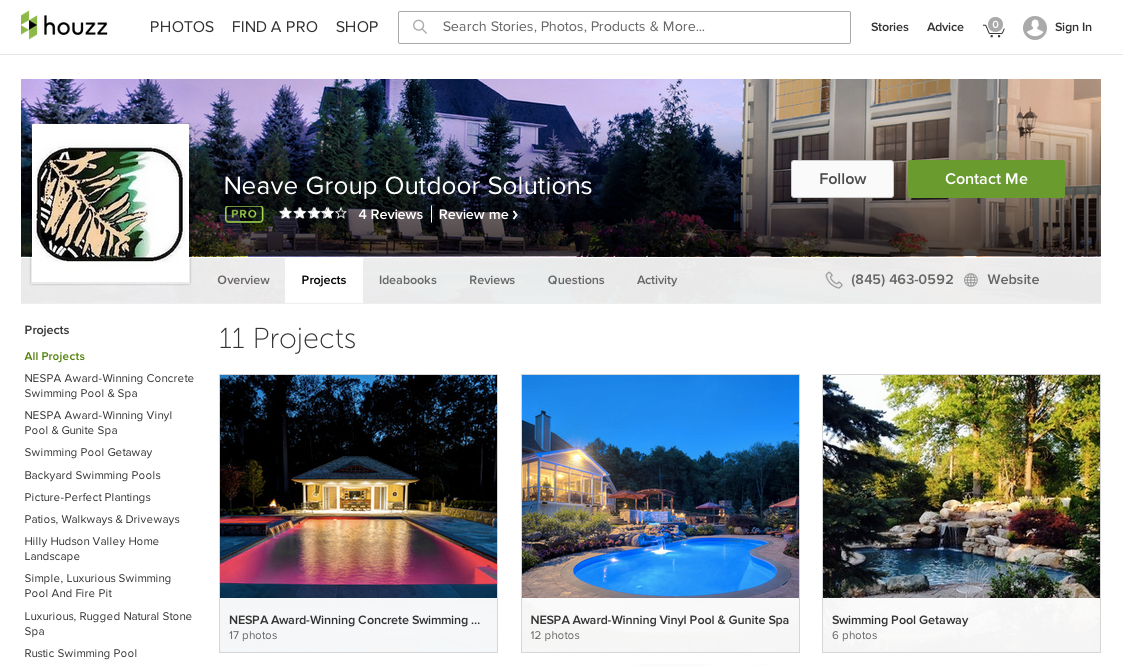**Detailed Caption**:

The interface displays a comprehensive profile for "Neve Group Outdoor Solutions Pro." At the top is a banner image labeled "Neve Group Outdoor Solutions Pro" with a distinct green 'Pro' symbol, rated four out of five stars based on reviews, accompanied by the prompt "Review me." 

On the far left, there's a logo depicting a forest. Below this, a picturesque photo showcases a house's backyard filled with lush trees, possibly including an interior glimpse. Adjacent to the logo, there are social connectivity buttons: "Follow" and "Connect Me," the latter highlighted in a green box.

Below this section, several navigation tabs are listed: Overview, Projects, Idea Books, Reviews, Questions, and Activity. 

A contact segment includes a phone icon followed by the number 845-463-0592, and a web icon indicating there is a link to the company's website.

Under the projects section, it mentions "11 projects" with accompanying images: 
1. A backyard pool with an adjacent pool house.
2. Another backyard scene featuring a well-designed patio.
3. A rock formation creating a waterfall effect into a pool with a surrounding forested area.

On the far left of the interface is a detailed project list under the heading "Projects" and "All Projects," enumerating the specific ventures completed by the company.

The header area includes a house icon with a logo resembling a green Triforce made up of three green triangles. To the right of this icon, navigation options read "Photos" and "Find a Pro," followed by a search bar with a magnifying glass icon labeled "Search stories, photos, products, and more." Additional menu items include "Stories," "Advice," a shopping cart icon, and a user avatar within a circle with the option to "Sign In."